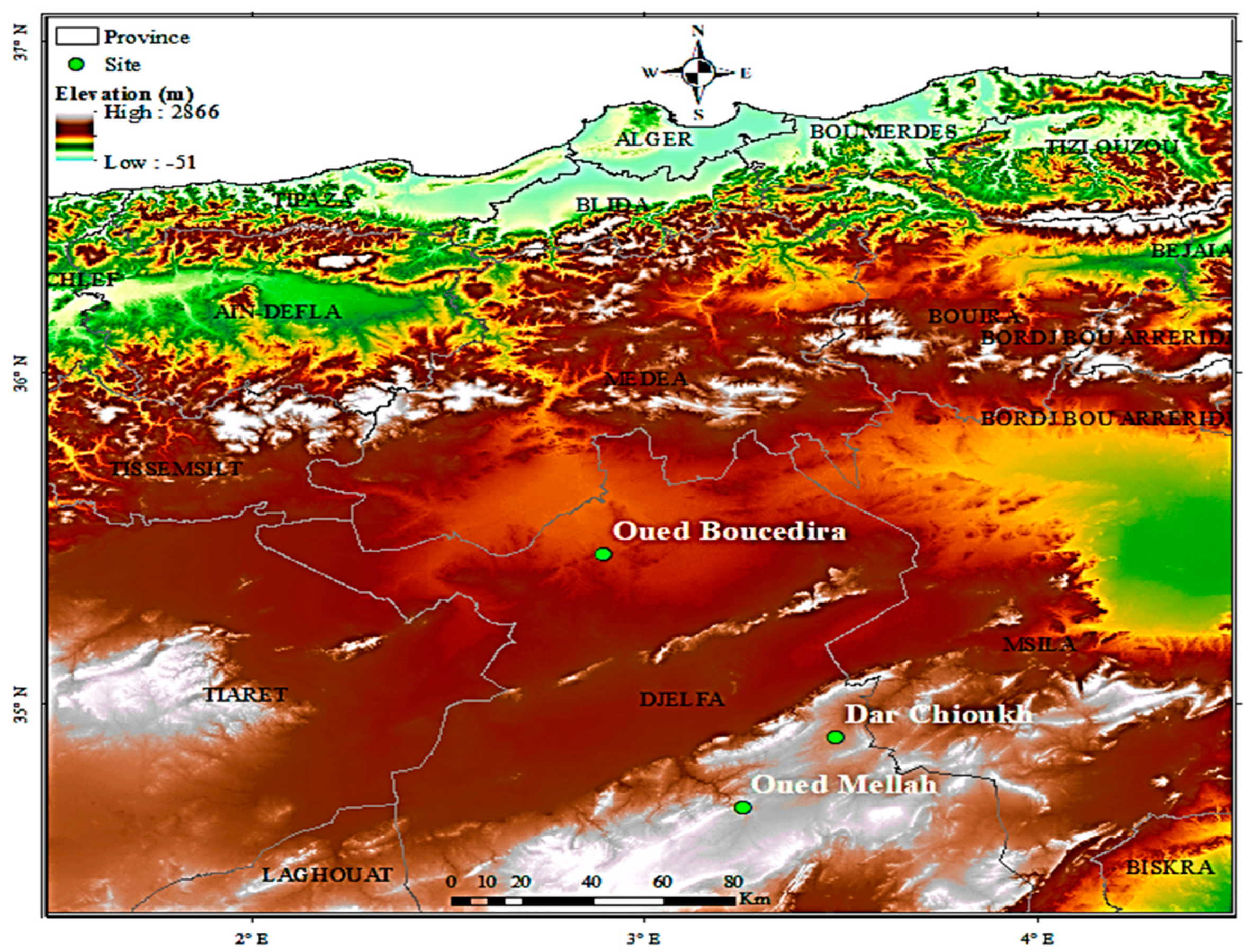This image is a detailed relief map of Algeria, located in the northern part of Africa, showcasing various regions marked by color-coded elevations and boundaries. The map features squiggly gray lines outlining provincial borders, highlighted by a white line for each province, and green dots signifying sites of interest. A compass rose at the top center indicates directions (north, south, east, west) with black and white points. The color scheme of the map ranges from deep red in the lower central area, indicating the highest elevation of 2866 meters, to neon green-blue in the top, representing the lowest elevation of minus 51 meters. Green areas dominate the coastal regions below the Mediterranean Sea, with patches of green also present in the middle-right section of the map. There is significant overlap and interspersion of colors (green, yellow, red, white) over the text, making the map intricate. Additionally, a legend in the top left corner provides information on provinces, sites, elevation, and color-coded high and low areas. At the bottom, a black and white scale bar labeled from 0 to 80 kilometers helps gauge distances. The map integrates multiple elements into a vivid, multi-colored visual representation of Algeria's diverse topography.